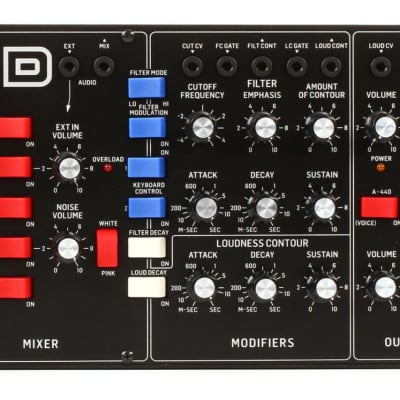The image showcases a detailed control panel against a black background, presumably for audio or sound manipulation. On the left side, there are five red switches arranged vertically. Adjacent to these switches are two silver knobs, labeled "EXT IN VOLUME" and "NOISE VOLUME." At the top-left corner, there are two black circular outlets or jacks, and a white letter "D" is visible nearby. Below these elements, the word "MIXER" is written in white text.

To the right of these controls, there is a column with one red switch above a label that mentions "OVERLOAD." Further right, another column features four blue buttons labeled "FILTER MODE," "LOW," "HIGH," and "FILTER MODULATION," followed by two white buttons labeled "KEYBOARD CONTROL" and "FILTER DECAY."

The central section contains nine silver dials arranged in a grid of three rows and three columns. These dials are labeled with terms related to audio modifiers such as "CUTOFF FREQUENCY," "FILTER EMPHASIS," "AMOUNT OF CONTOUR," "VOLUME," "ATTACK," "DECAY," "SUSTAIN," and "LOUDNESS." At the bottom of this section, the word "MODIFIERS" appears in white text.

On the right side, the panel continues off the edge of the image but displays another section with a silver dial at the top, a red switch in the middle, and another silver dial near the bottom, partially labeled "Q OU," with the last letters cut off.